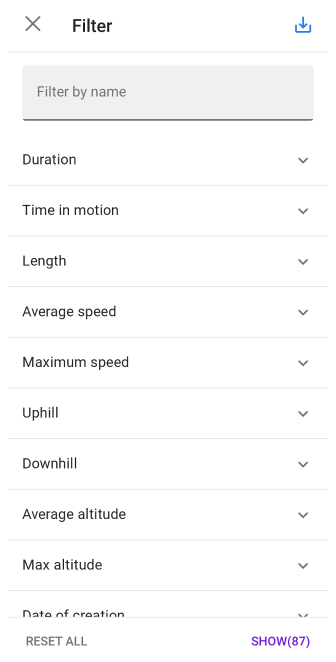Screen capture of a mobile application interface showcasing a filtering feature. The image highlights the top header of the page, featuring an "X" button on the upper left side, followed by the word "Filter" in black text. On the upper right corner, there's a blue download icon depicted as a downward-pointing arrow. Directly below, a light gray text box displays the words "Filter by Name."

Beneath this, the interface presents several dropdown options arranged in ten rows, each with a dropdown arrow on the right side. These options include:
1. Duration
2. Time in Motion
3. Length
4. Average Speed
5. Maximum Speed
6. Uphill
7. Downhill
8. Average Altitude
9. Max Altitude
10. Date of Creation

These options are neatly laid out, providing a structured and detailed way to filter various parameters within the application.